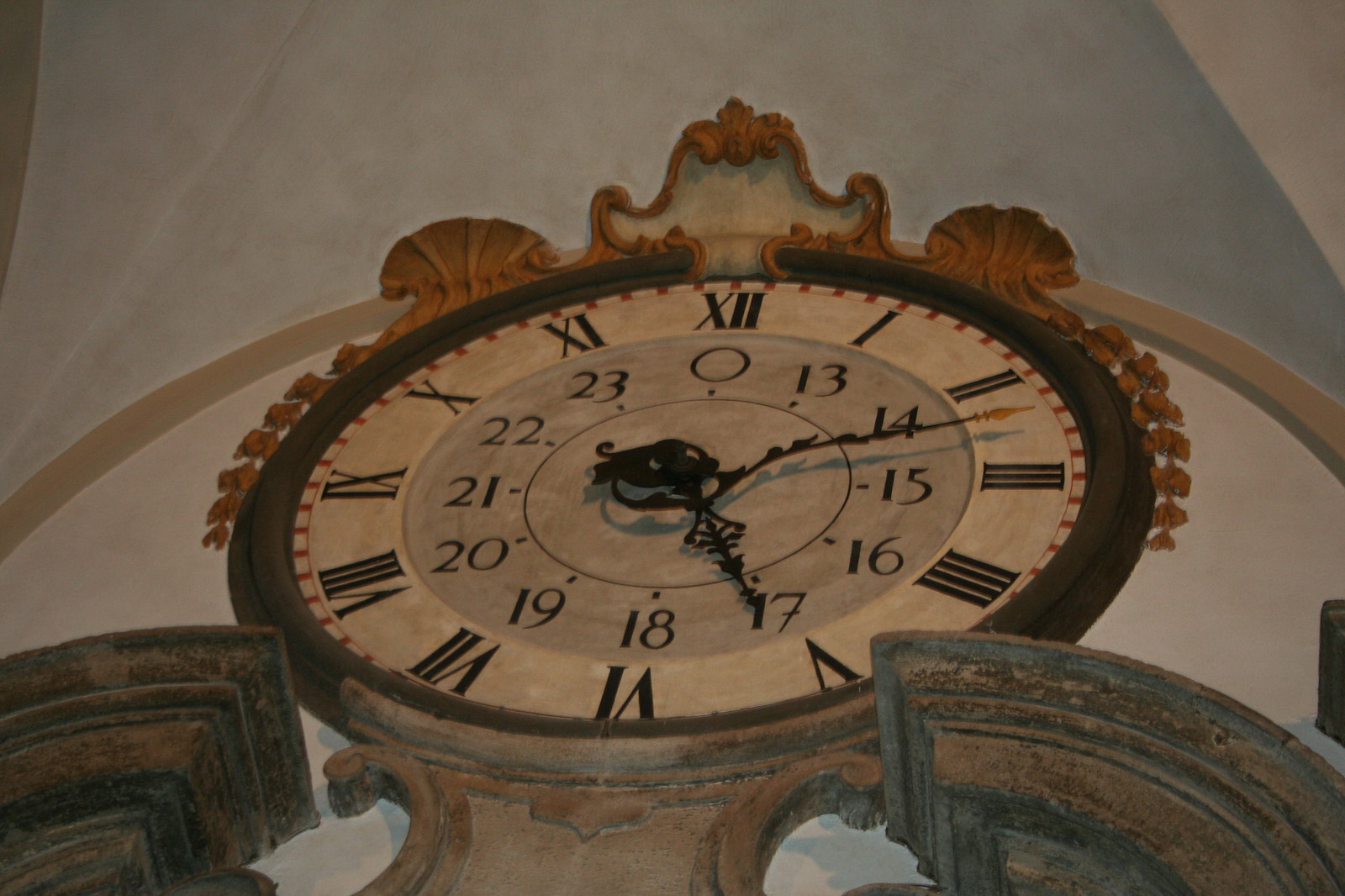This photograph features an ornate wall clock with a unique dual-layered display. The clock itself is circular and employs Roman numerals to denote the hours along the outer edge. The hour and minute hands are elegantly curved and intricately decorated, reflecting a classical design. Within the outer circle lies an inner ring marked by Arabic numerals, which appear to indicate a 24-hour scale, adding a layer of complexity to the timekeeping. The clock is mounted on an ivory-colored wall, above which is an ornately decorated plaster ornament resembling a shell. This plaster decoration is a dull orange hue, providing a striking contrast to the subtle background and enhancing the overall aesthetic appeal of the display.